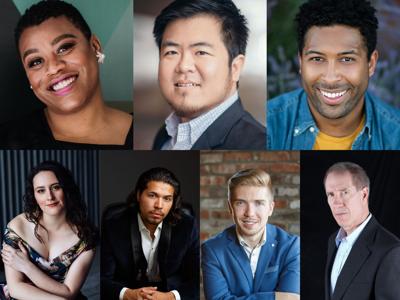This image is a collage consisting of seven portrait photographs of diverse individuals, arranged in a grid with three images on the top row and four on the bottom row. 

In the top left, there is a smiling woman of color with short hair and large earrings, tilting her head slightly to the left. In the center of the top row is an Asian man with short black hair, a slight smile, and a cautious expression. He wears a blue and white checkered shirt under a dark suit jacket. The top right image features a male person of color with short hair and a beard stubble. He has a bright, happy smile and is dressed casually in a yellow t-shirt and blue denim-style shirt.

The bottom row starts on the left with a Caucasian woman with long brown hair, smiling softly with her arms crossed. She is wearing an off-the-shoulder dress. Next to her is an Asian man with long hair and stubble, dressed in a dark jacket and white shirt, with a professional demeanor in a dark background. The third image on this row is of a Caucasian man with short blonde hair, smiling against a brick background while wearing a light blue suit jacket and white shirt. The final image on the bottom right features an older Caucasian man in his 50s, with a serious expression. He wears a white shirt and dark suit jacket, set against a dark background.

Each person in the collage is facing the camera, suggesting they are posing for professional headshots.